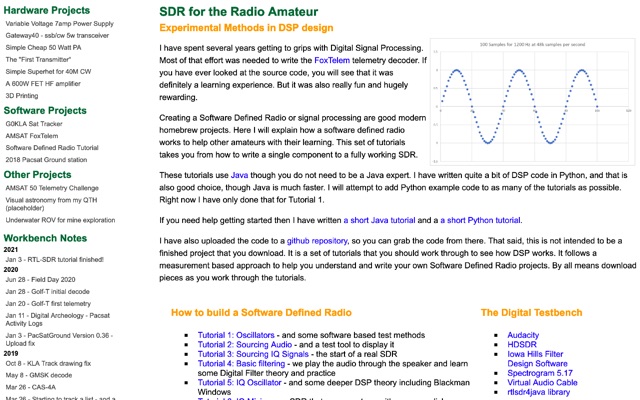The image depicts a detailed, text-heavy poster on a solid white background, styled to appear as if printed from a computer screen. The layout prominently features multiple sections organized by thematic headers in green text along the left side. These include "Hardware Projects" with seven lines of text, detailing topics like power supply and a 50-watt PA; "Software Projects" with four lines of text mentioning a sat tracker and a software-defined radio tutorial; "Other Projects" with three lines of text; and "Workbench Notes" listing projects and notes from 2021, 2020, and 2019.

In the upper right corner, there is a small graph resembling a dotted sine wave with an unreadable black title and indistinguishable x and y axes. 

The central portion of the poster is dominated by a title in green that reads "SDR for the Radio Amateur," followed by a subheading in orange, "Experimental Methods and DSP Design." Beneath this are four paragraphs of left-aligned text discussing various aspects of the subject, including mentions of a "Foxtelum telemetry decoder." Several words within these paragraphs are highlighted in blue.

At the bottom center, a section titled "How to Build a Software-Defined Radio" in orange includes black bullet points with some highlighted blue links. To the right is another section with an orange subheading, "The Digital Test Bench," also featuring bullet points with some blue highlights. The overall style is minimalistic with sparse illustrations, focusing heavily on informational content.